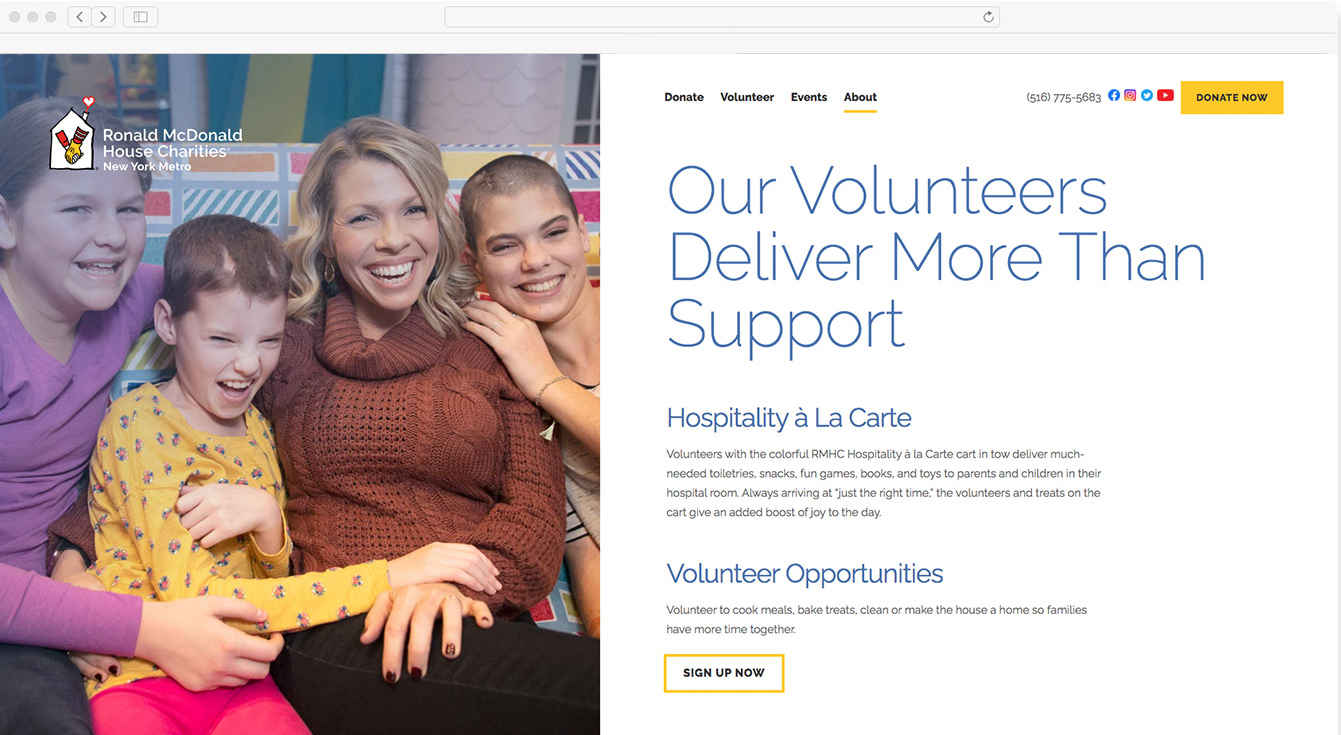A screenshot of a website displayed on a computer screen. The website has a grey navigation bar at the top, featuring a probable search button centered and three dots accompanied by two navigation arrows (one pointing left and the other right) at the right side. Below the grey bar, the webpage has a predominantly white background. 

On the left, occupying almost half of the page, there's a prominent image featuring the Ronald McDonald House Charity of New York, with the name inscribed in white ink. The image shows a woman sitting with three smiling children. 

On the right side of the webpage, there are several menu options listed in black ink: Donate, Volunteer, Events, and About. The 'About' option is highlighted with a yellow underline. Below the menu, a blue tagline states, "Our volunteers deliver more than support." Further down, yet also in blue ink, is the text “Hospitality à la Cartier.”

There are sections of text in black ink that appear less legible in the screenshot, and the phrase "Volunteer Opportunities" is noticeable in blue ink. Near the bottom of the page, there's a textbox with a yellow outline containing the call-to-action "Sign up now" in black ink against a white background.